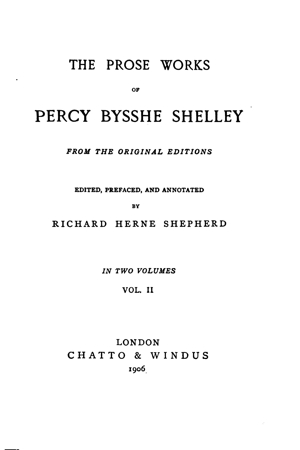The image is a title page from a book with a plain white background. At the top, in all capital letters and medium-sized black font, it reads "THE PROSE WORKS." Directly below, in a smaller font, is the word "OF." Following this, in a larger and bolder font, the name "PERCY BYSSHE SHELLEY" is prominently displayed. Below Shelley's name, in a smaller italicized font, it states "From the Original Editions." Further down, in even smaller print, it mentions "Edited, Prefaced, and Annotated by," followed by the editor's name, "RICHARD HERNE SHEPHERD," in larger font. Underneath this, in italicized print, it notes "In Two Volumes," and non-italicized, "Volume Two." At the very bottom, it lists the publication details: "London: Chatto and Windus, 1906."